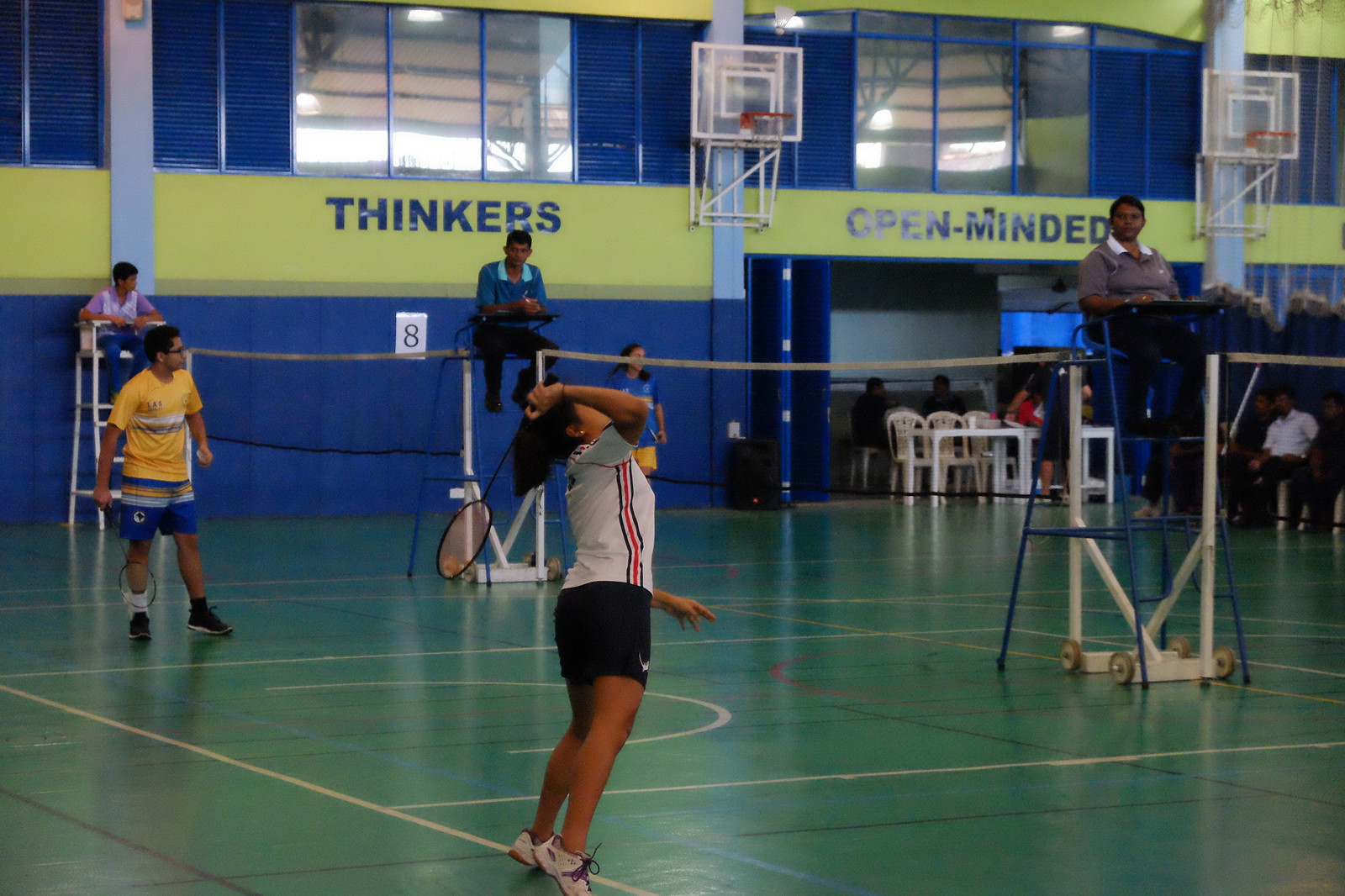In this vibrant indoor sports arena, predominantly featuring the colors green, blue, and yellow, a dynamic scene unfolds on the green-painted gym floor with white lines marking badminton courts. The walls are blue and adorned with a yellow stripe at the top, displaying the words "THINKERS" and "OPEN MINDED" in bold blue letters. 

The image captures three simultaneous badminton games in action. A woman positioned to the right is poised to hit the shuttlecock over the net, while other players, a mixed group of young men and women, are immersed in their matches. Among the players is a girl in the foreground wearing a white t-shirt with red and blue stripes, black shorts, and white shoes, gripping a badminton racket. Behind her stands a young man in a yellow t-shirt, black eyeglasses, and blue-yellow-white shorts, also ready with his racket.

Three referees are seen seated on chairs along the nets—each presiding over one of the three courts. The vivid scene is further complemented by white chairs set off to the side and basketball hoops visible near the top right.

The diverse palette of colors extends to various elements in the image, including apparel and equipment, featuring hues of yellow, black, white, red, orange, pink, and light blue. The overall composition highlights a lively and engaging sports event, capturing the essence of indoor athletic competition.